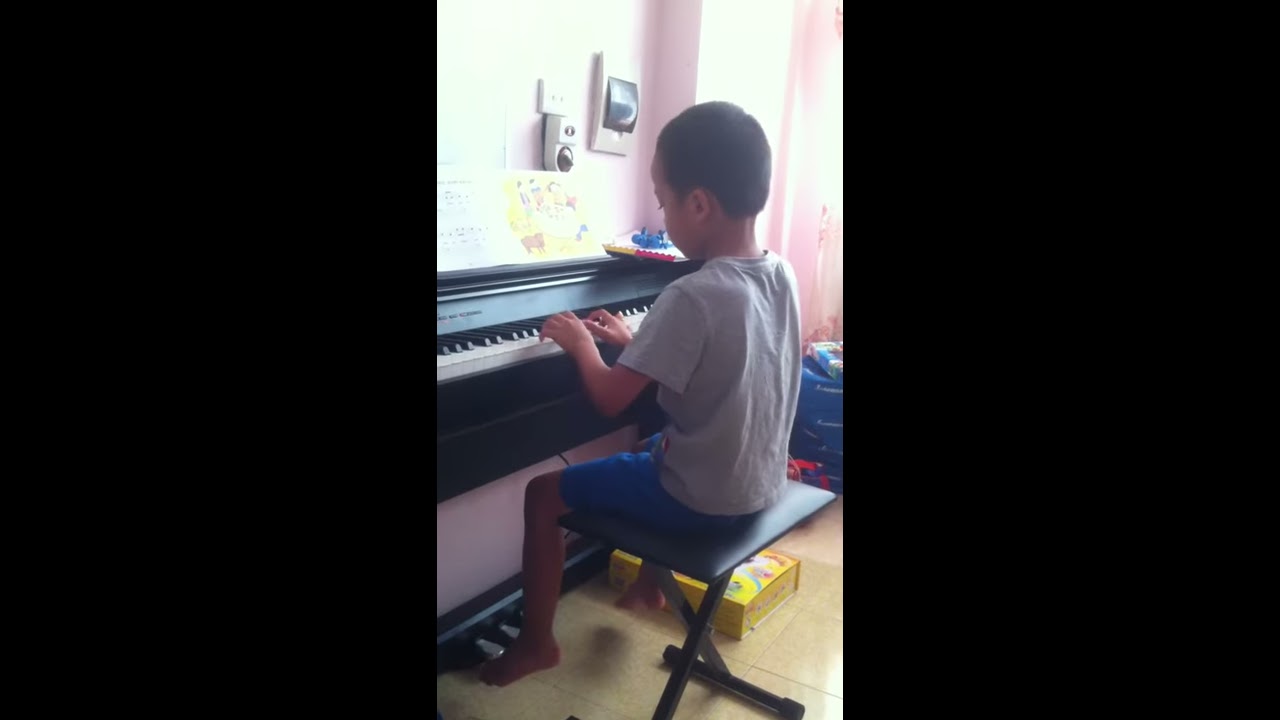The image shows a young child, identified as a boy with dark hair and slightly darker skin, deeply engrossed in playing a black piano. He is barefoot and sits on a black folding stool with a padded vinyl leather top. The child is dressed in light blue pants and a short-sleeved gray shirt. The piano features a book in front of him with a yellow page on the right and a white page adorned with various musical notes on the left. The scene is set in a room with light pink painted walls. Behind the piano, a light switch and a camera are mounted on the wall. On the floor, made of tile, next to the child's foot, a yellow box is visible. To the right side of the image, there is a short and low four-drawer piece of furniture.